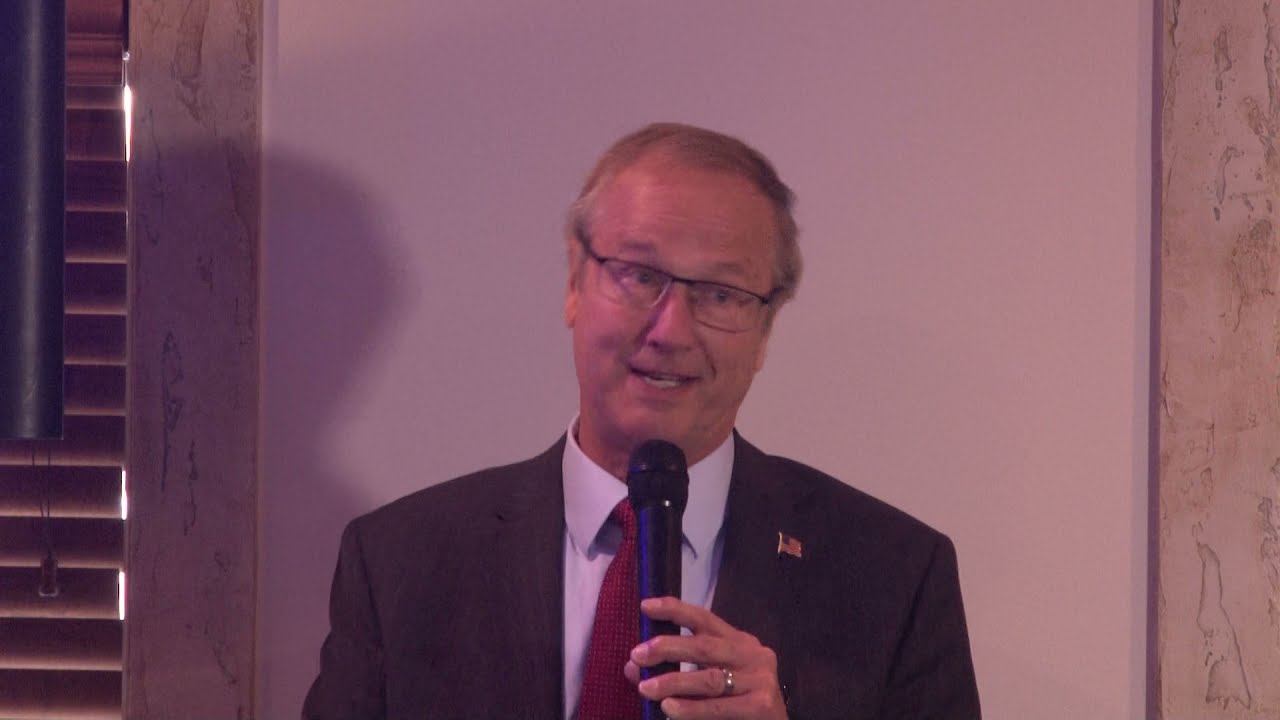The image captures an older white man in his 60s with short gray hair styled to one side, wearing rimless glasses and a gray suit jacket adorned with an American flag lapel pin. He is dressed in a light blue collared shirt complemented by a red tie. The man is speaking into a black microphone held in his left hand, which also bears a gold wedding band. He stands before a white wall, flanked by vertical rectangles of light gray marble. Toward the right of the image, there is a set of horizontal rectangular blinds covering a window, with a hint of wood grain visible. A black cylinder, potentially a cover for shade strings or a wind chime with a central string, hangs down on the left side of the image. The photograph shows the man from about mid-chest upwards, looking slightly to the right as he addresses an unseen audience.